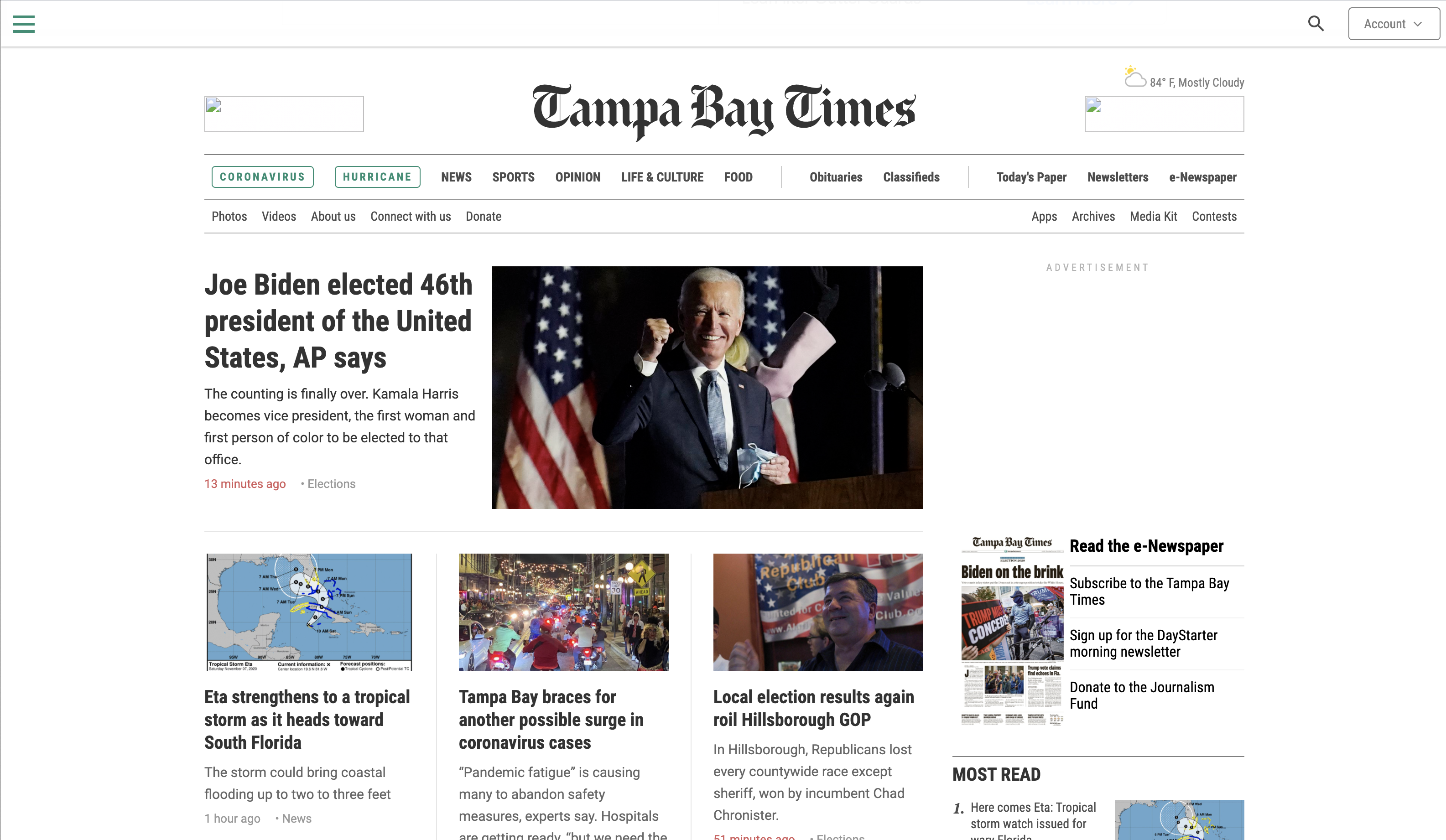The image is a screenshot of the Tampa Bay Times website. It has a clean design with a white background and black text. At the top center, the website's logo, "Tampa Bay Times," is prominently displayed. Beneath the logo, there is a navbar with various sections including "Coronavirus," "Hurricane," "News," "Sports," "Opinion," "Life and Culture," "Food," "Obituaries," and "Classifieds."

In the center of the image, there is a large photograph of Joe Biden with his fist raised in the air, flanked by two American flags. To the left of the photo, a headline reads, "Joe Biden elected 46th President of the United States, AP says. The counting is finally over. Kamala Harris becomes Vice President, the first woman and first person of color to be elected to that office."

At the bottom of the image, there are three rectangles displaying different headlines. The first rectangle features a map showing land and water, accompanied by the headline, "Eta strengthens to a tropical storm as it heads towards South Florida." The second rectangle shows an outdoor scene with a crowd of people and is headlined, "Tampa Bay braces for another possible surge in coronavirus cases." The third rectangle, depicting a man with an American flag behind him, has the headline, "Local election results, again, roll Hillsborough GOP."

To the far right of these rectangles, there is a section prompting users to “Read the e-newspaper” with options to subscribe and sign up for the service.